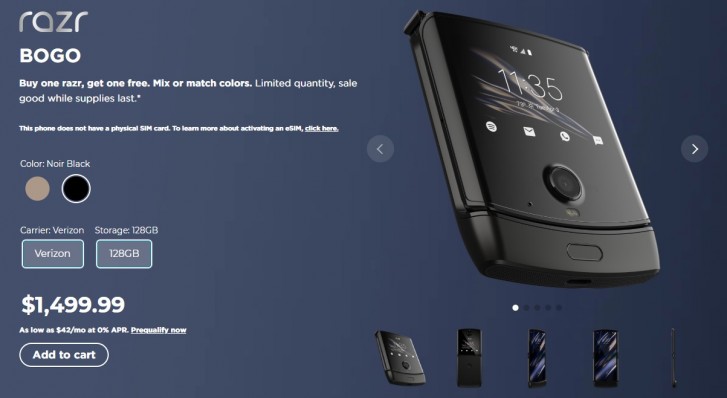The image features a promotional offer for the Razer phone model "R-A-Z-R." The sleek, foldable smartphone is showcased with a detailed advertisement highlighting the following points:

- **Headline:** "Buy One Razer, Get One Free" in bold, capital white letters.
- **Offer Details:** Mix or match colors, limited quantity available, and the sale is valid while supplies last.
- **Additional Info:** The phone operates without a physical SIM card. Instructions to learn more about activating an eSIM are provided with an underlined "click here" link.
- **Color Options:** Featured colors include tan and black. The selection in the image highlights the black color option with a white line around the black circle.
- **Carrier:** Verizon is specified as the carrier in a rectangular label.
- **Storage:** The phone has 128 GB of storage capacity.
- **Pricing:** The device is priced at $1,499.99. Financing options include payments as low as $42 per month at 0% APR, with a "Pre-Qualify Now" option available.
- **Action Button:** An "Add to Cart" button is prominently displayed.
- **Visuals:** At the bottom of the image, the phone is shown in both its open and closed states to illustrate its foldable design.

The overall presentation is designed to attract potential buyers with a clear, detailed description, emphasizing the unique selling points and promotional offer.